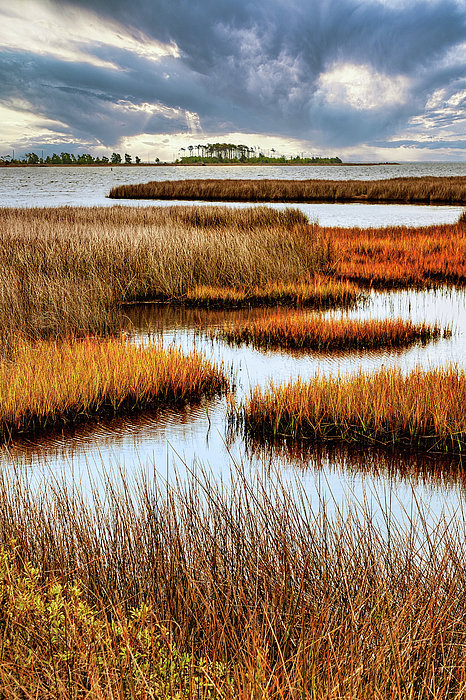The photograph showcases an expansive wetland area characterized by multiple small patches of elevated land interspersed within a larger body of water. These patches are densely covered with tall yellow and brown grasses and reeds. Scattered throughout are several deep-looking puddles filled with brownish water. In the distance, a larger bluish-gray body of water stretches towards the horizon, where a flat strip of land is visible. This distant land is densely populated with various green trees and a small clump of palm trees. The sky above is a light blue adorned with dark, non-stormy clouds that allow sunbeams to pierce through, casting a golden hue over the scene—suggesting that the photograph was taken near sunset. The overall composition creates a sense of a serene, undisturbed natural landscape.